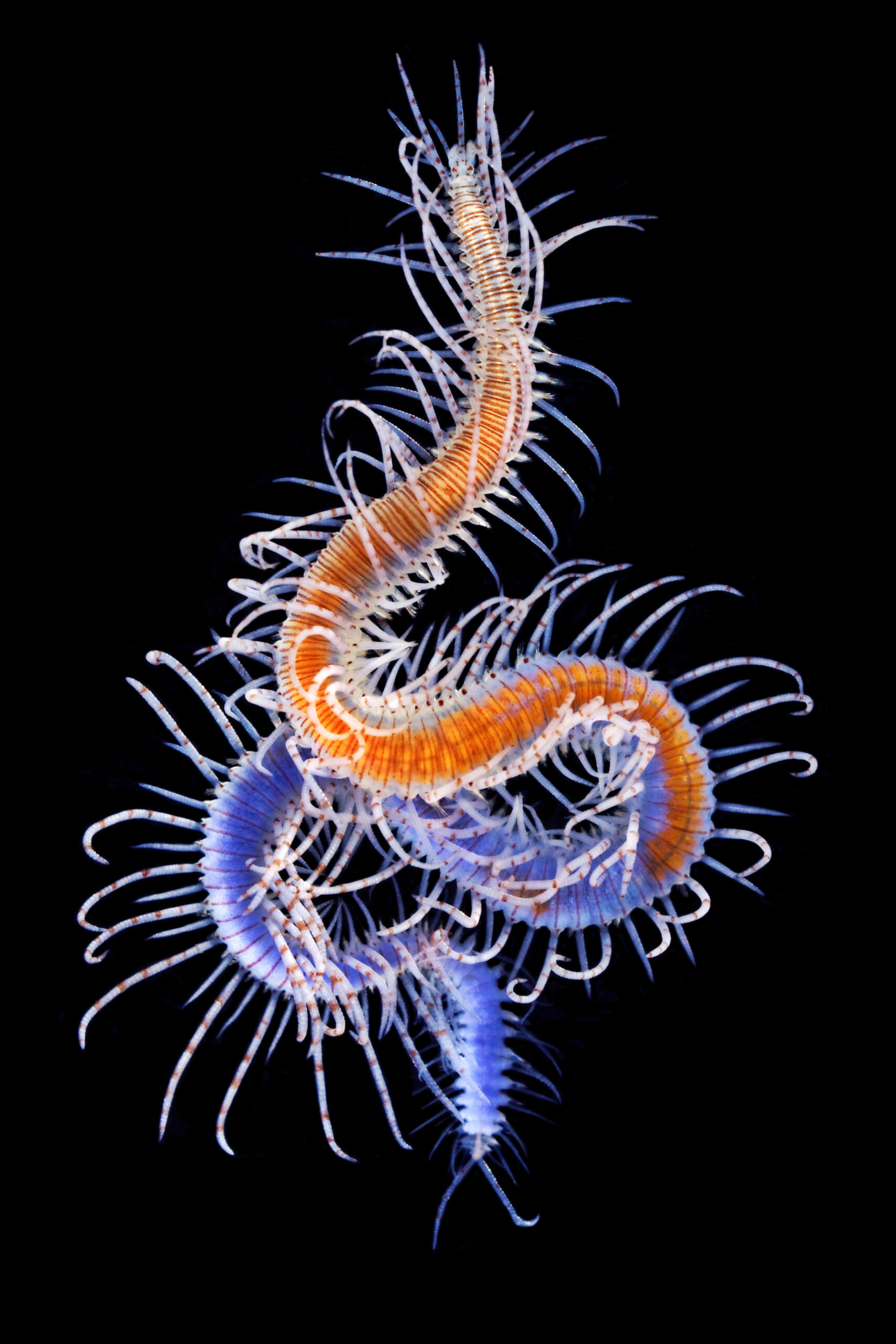In this highly detailed, up-close image, likely a professional photograph or a microscopic view, we observe a striking centipede-like creature set against a stark black background. Dominating the frame, the creature seems either to be one single entity with intricate coloration or possibly two intertwined. The segmented body displays a vivid gradient, with the lower part showcasing a light purplish-blue hue, transitioning to an orange-tinted section. Its hundreds of whiskery white legs emerge in delicate, horizontal patterns, some featuring red stripes. The only colors present in this image are the purplish-blue, orange, and white of the creature, creating a stark contrast against the monochrome backdrop. No other objects or text distract from the focus on this fascinating, many-legged organism.